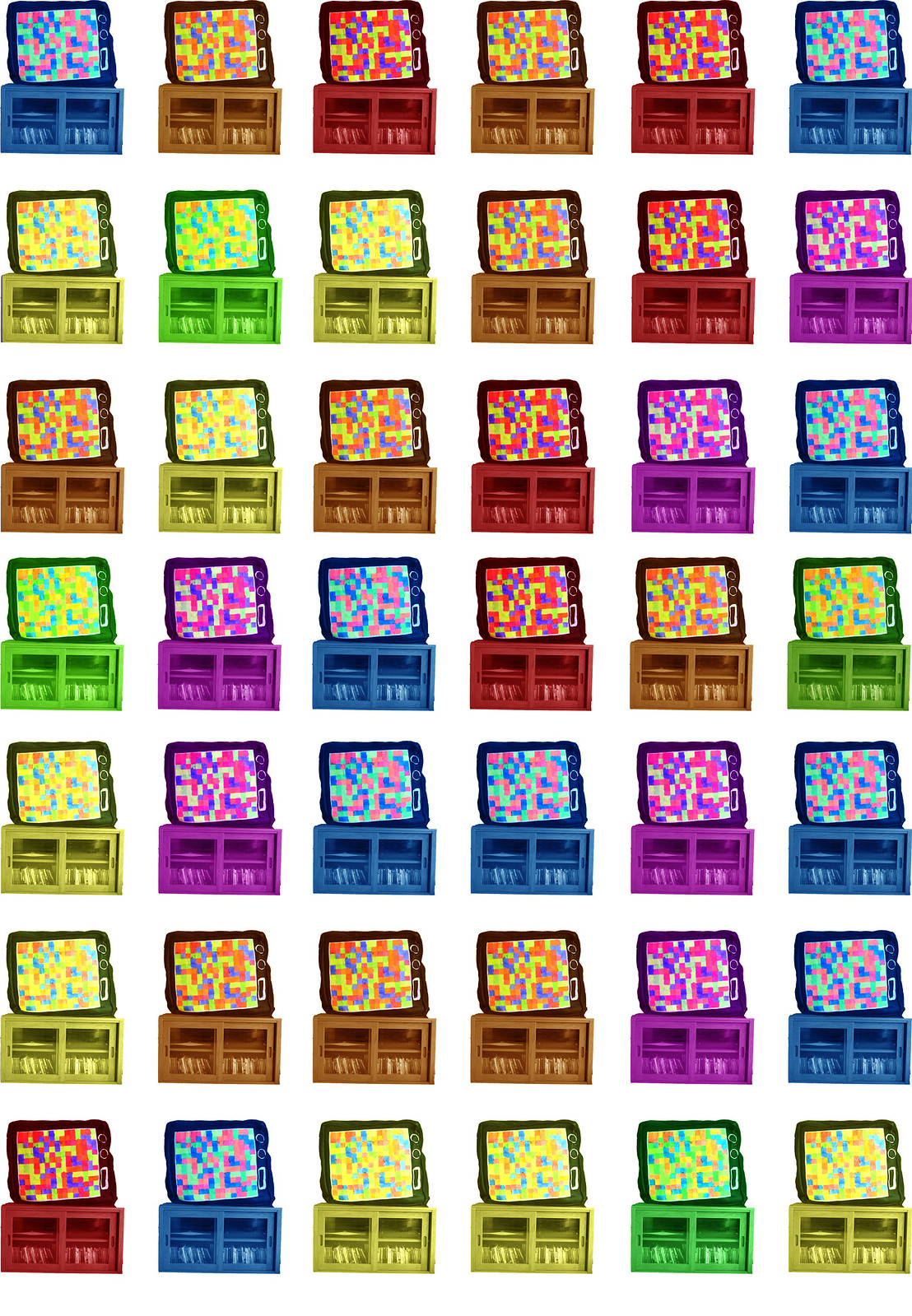The image showcases a vibrant, pop-art inspired artwork featuring an array of colored TVs atop corresponding TV stands, arranged in a precise grid of six columns by seven rows. Each TV stand exhibits a distinct hue, including blue, yellow, green, purple, and brown. The TVs display pixelated screens with varied collages of colors: light blue and pink on the blue TVs, red, yellow, and purple on the red TVs, purple and pink on the purple TVs, green and orange on the green TVs, and yellow, red, and blue on the yellow TVs. The artistic piece resembles a wall of clip art, depicting cartoony analog televisions on wooden stands with clear-doored shelves, often resembling DVD collections. The repetitive, tinted images create a colorful, orderly, and striking visual effect in the style of classic pop art.